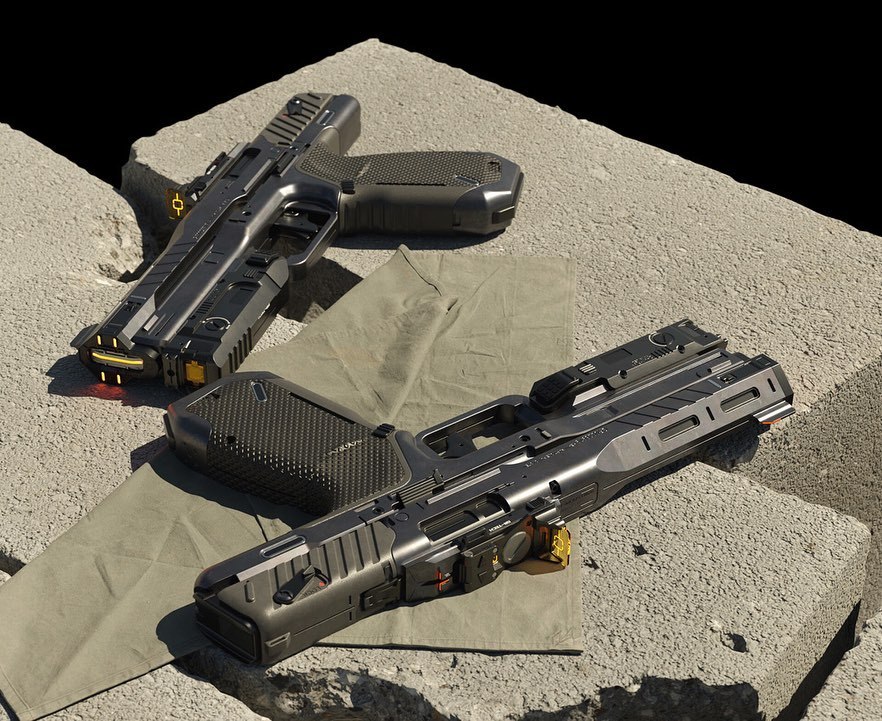In this color photograph, we see two identical pistols, which appear to be laser tag guns or tasers, laid out on light gray cinder blocks. The photograph captures these dark gray, almost black, guns glistening slightly under sunlight. One gun, positioned closer to the viewer, points to the upper right with a square barrel and a textured brown grip; it features an attachment beneath the barrel that could potentially be a laser sight. This gun rests partially on a folded gray cloth. The second gun, behind the first, points to the lower left. Both guns have a yellow light source where the muzzle would be. The background of the image is a plain black, enhancing the contrast with the cinder blocks and the guns.